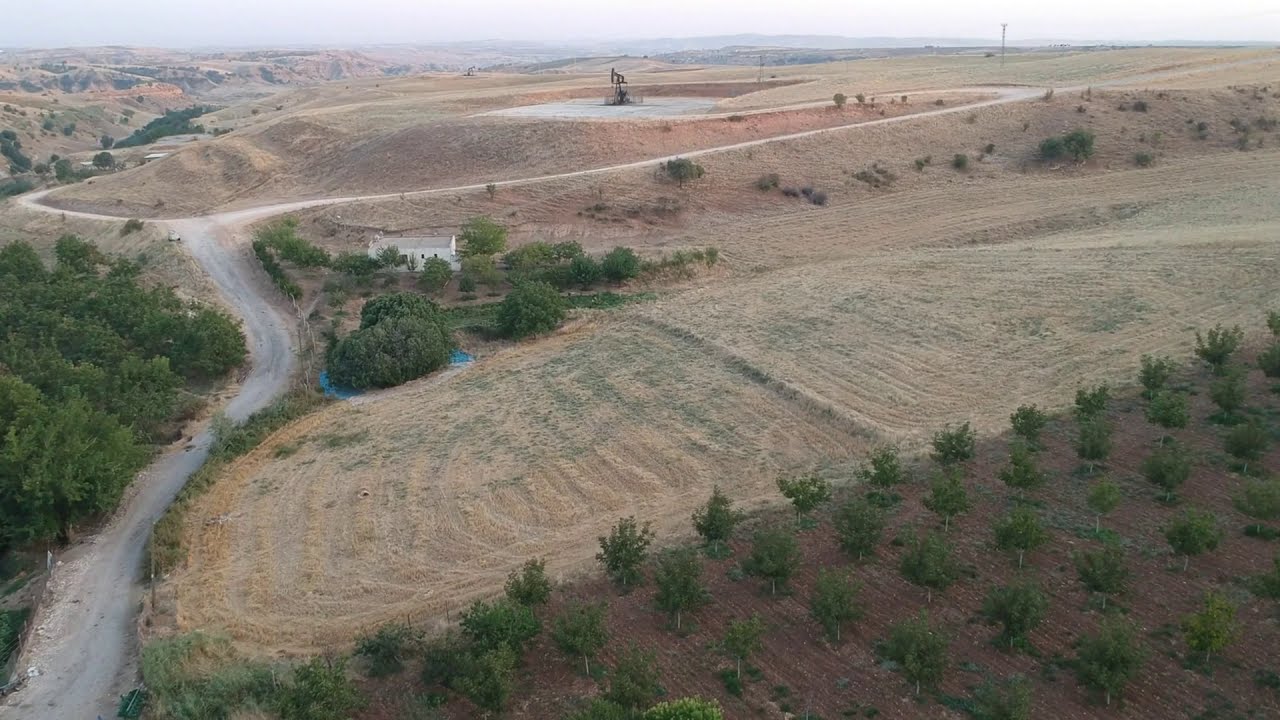The image captures a rural landscape, likely in winter, as evidenced by the predominantly brown ground and sparse greenery. Set against an overcast sky, a small white house surrounded by green trees stands out in the mid-ground. The land appears to be farmland, possibly an orchard or vineyard, given the neat, orderly rows of what might be apple or orange trees, or perhaps olive trees. There are winding dirt roads crisscrossing the scene, suggesting limited vehicular access. In the background, a significant crane or oil derrick, surrounded by concrete or gravel, hints at possible oil extraction activities. Sparse green bushes and small evergreens dot the otherwise barren terrain, which has either been freshly tilled or shows signs of recent logging activities.